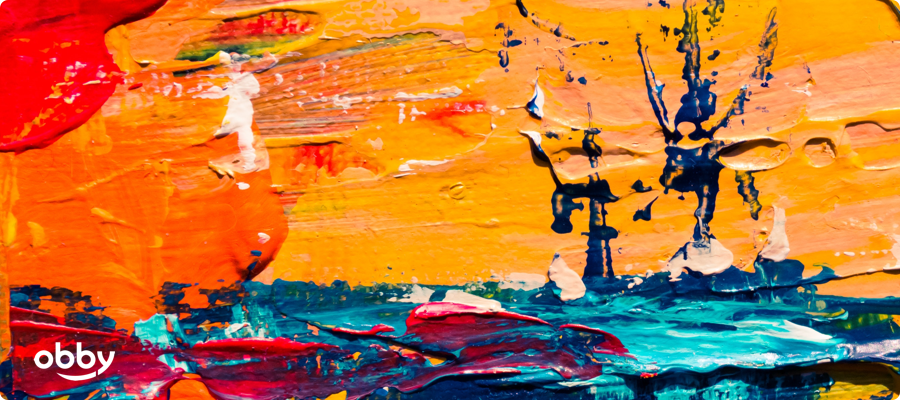This vibrant and textured painting on a rectangular canvas board uses a striking blend of acrylic paints to create an abstract seascape. A thick base layer of yellow dominates the upper sky, transitioning into streaks and splatters of orange, red, and occasional blue on the left-hand side. These colors create a dramatic, warm atmosphere. The lower portion depicts a tumultuous sea in shades of turquoise, dark blue, dark red, and hints of yellow, mimicking the fluid motion of waves. A dark blue painted boat with two upright posts, almost resembling sails, is a central focal point. The paint application is thick and textured, suggesting the use of a palette knife, further emphasizing the painting’s tactile quality. Notably, blue splatter marks dot the upper right yellow sky, adding to the dynamic composition. The bottom left corner features the white text "OBBY," adding an element of intrigue to the artwork.